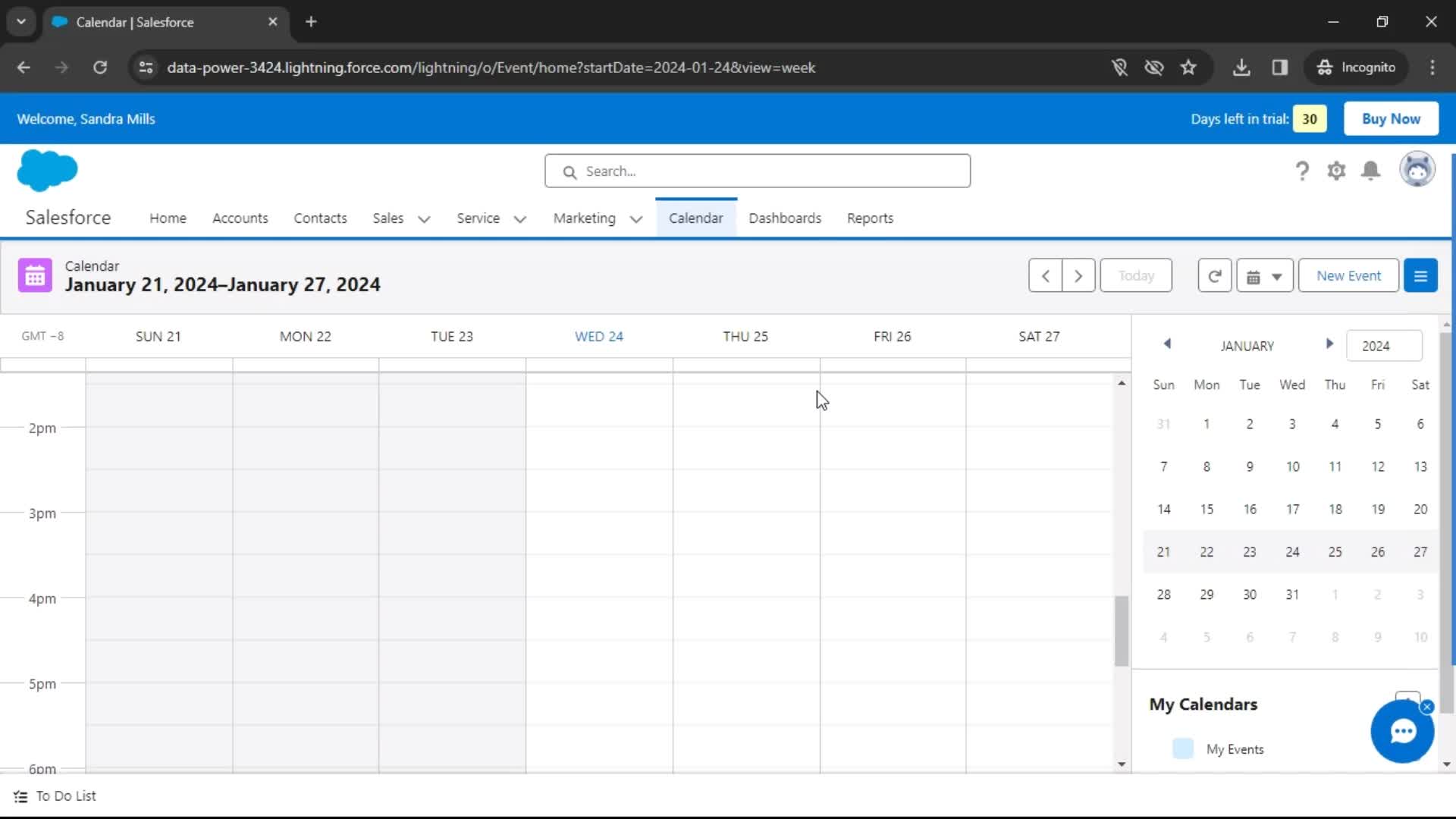This screenshot depicts a user's calendar interface within the Salesforce platform. At the top, the tab is black and labeled "Calendar - Salesforce." The address bar displays the following URL: `data-power-3424.lightning.force.com/lightning/o/event/home?startDate=2024-01-24&view=week`.

Beneath the address bar is a blue banner with white text that reads, "Welcome Sandra Mills. Days left in trial: 30," accompanied by a "Buy Now" button. 

The main calendar view spans the week from January 21st, 2024, to January 27th, 2024. The calendar is organized with columns for each day and rows indicating time blocks ranging from 2 PM to 6 PM. 

On the right side of the interface, there is a smaller inset monthly calendar displaying January 2024. The week of January 21st through January 27th is highlighted in gray.